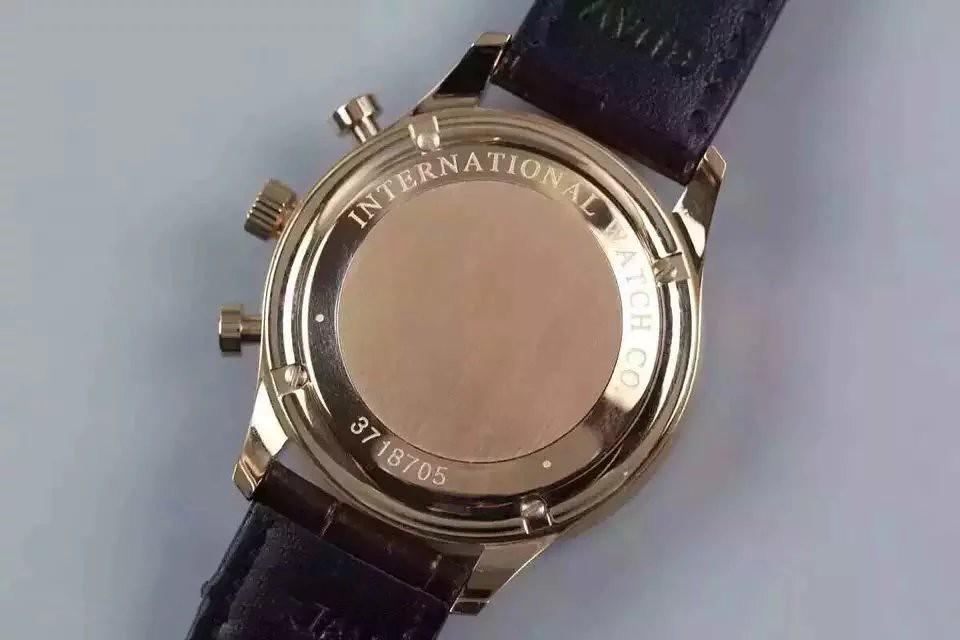The image depicts the back of a gold or brass-colored watch, centrally framed against a white, hard surface. Shadows subtly cast beneath the watch indicate it's placed on a smooth, countertop-like surface. The watch back is round, with the words "International Watch Co." etched at the top edge. At the bottom, a serial number "3718705" is also etched. On the left side of the watch, there are three circular dials—one used for winding and setting the time, and two nubs likely for operating stopwatch functions. The watch features a black leather wristband visible at both the top and bottom, with some embossing or engraving on the upper part of the band.